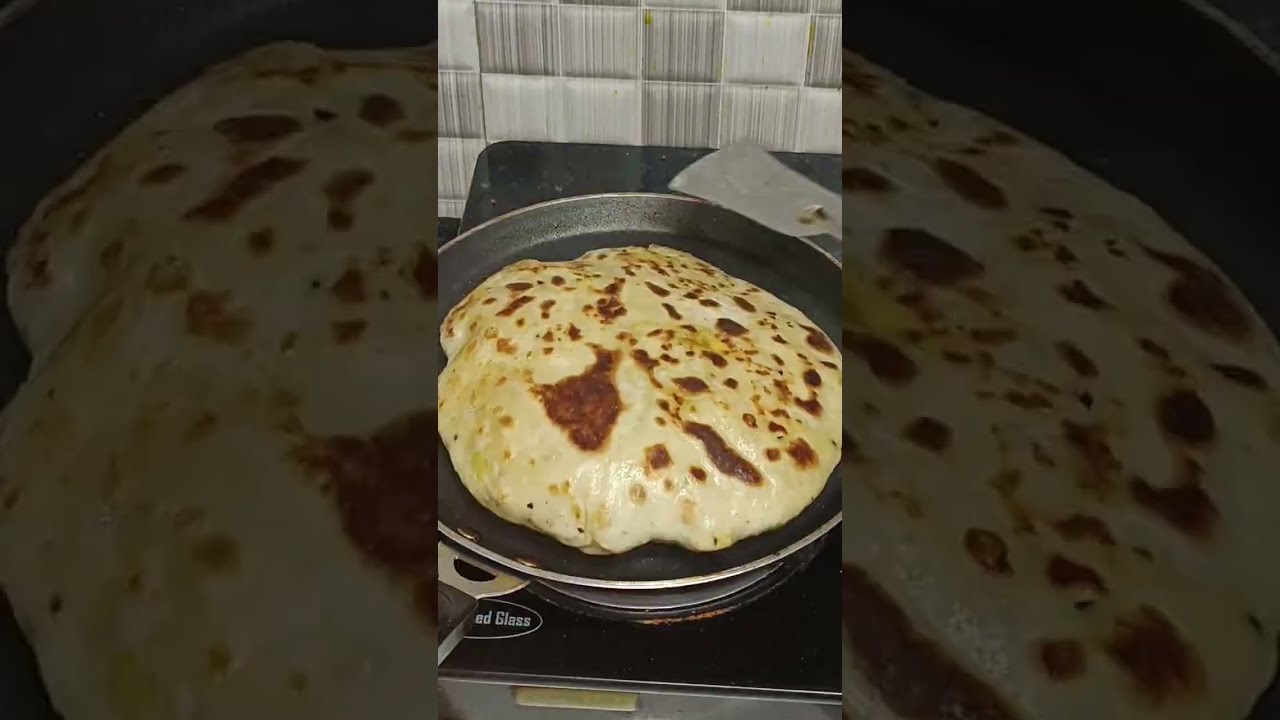The image centers on a vertical cell phone photograph, surrounded by a background that is a zoomed-in and faded version of the same scene. In the main photo, a piece of bread or a pancake, puffed up and slightly charred with brown spots, is being cooked in a large black, shiny frying pan on a stove top, which could be either gas or electric. The head of a metal spatula rests above the back end of the pan, suggesting that someone is in the process of cooking. The wall behind the stove is lined with square gray tiles, some featuring vertical stripes. The puffy, overcooked appearance of the bread or pancake indicates that the heat might be too high. Overall, the scene captures the essence of a kitchen moment, mid-cooking process.